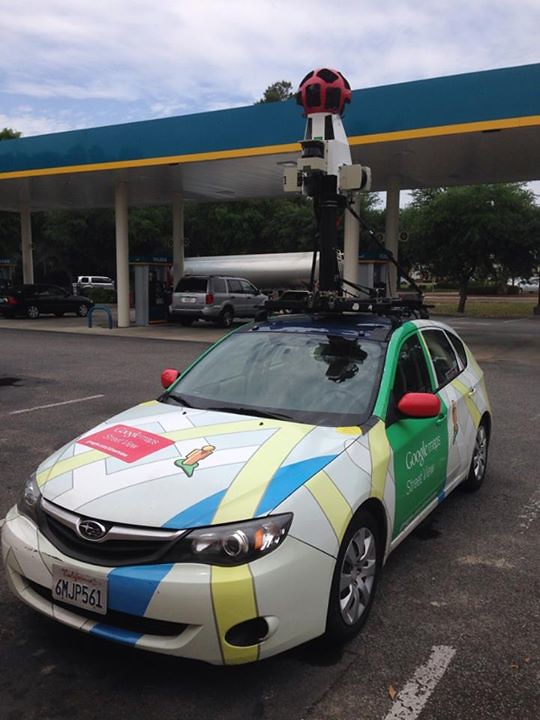This daytime photograph captures an outdoor scene featuring a parking lot in the foreground and a gas station in the background. The gas station is characterized by its distinctive green roof with a yellow border, and there are multiple cars, including a silver minivan, parked at the gas pumps. Notably, a gas tanker truck is also visible.

Dominating the foreground is a four-door white vehicle known as the Google Maps car. The car is adorned with a multicolored wrap that resembles roadways, featuring white, yellow, and blue lines. The driver's side door is painted green with the word "Google" visible on it, and the back of the car sports a red side mirror. Atop the vehicle sits an elaborate camera system mounted on a metal stand, crowned with a sphere-like object that appears similar to a soccer ball, characterized by an orange base and black square patterns. The clear sky with scattered clouds adds to the daytime ambience of the photograph.